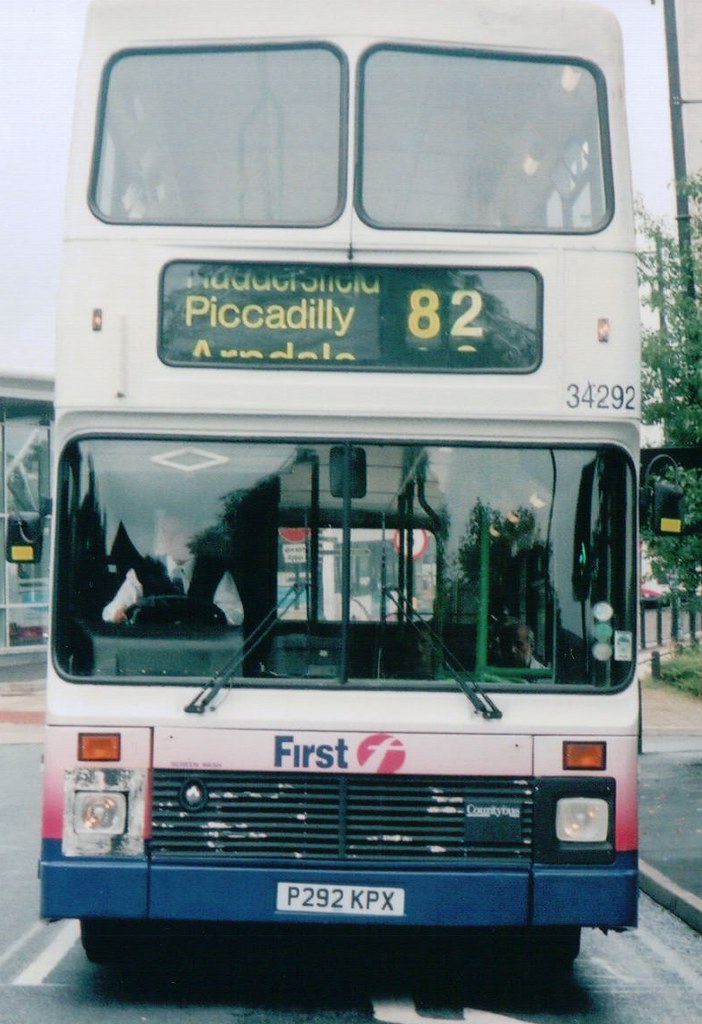This photograph captures the front view of a vintage white double-decker British bus on the road. The bus prominently features the destination sign "Piccadilly 82" written in yellow against a black background above the windshield. The driver, seen through the windshield, is wearing a black vest over a white button-down shirt, although a glare obscures his head slightly. The bus displays the word "first" above its flat front, indicating the brand. The license plate reads "P292 KPX" in black text, and the bus number "34292" is also visible on the right-hand side of the bus. The bus is framed by a minimal background, showing a glimpse of buildings, trees with green leaves, and partially another bus, emphasizing the vehicle itself in the foreground. The lower part of the bus, near the lights, features subtle pink and blue accents, making the overall scene a nostalgic glimpse of classic British transportation.